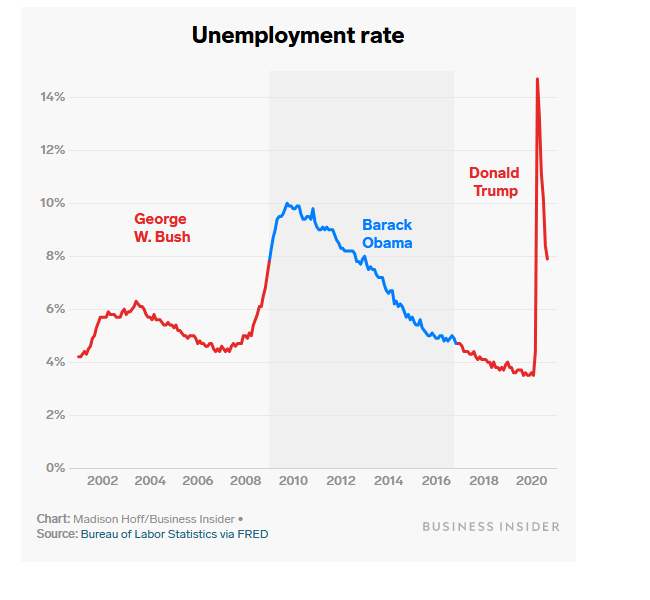The image displays a detailed line graph illustrating the unemployment rate from 2002 to 2020, segmented by presidential terms. At the top center of the graph, the title "Unemployment Rate" is inscribed in black text over a white or light gray background. The y-axis, labeled in percentage, ranges from 0% to 14% in 2% increments, while the x-axis is marked with years, starting from 2002 and progressing to 2020 in two-year intervals.

Text at the bottom left of the graph indicates its source: "Chart by Madison Hoff, Business Insider. Source: Bureau of Labor Statistics via FRED," and the bottom right corner bears the Business Insider logo in darker gray. The graph itself is central in the image.

The timeline begins with a red line representing George W. Bush’s presidency from 2002 to 2008, showing unemployment rates fluctuating between 4% and 6%, peaking occasionally near 7%. A vertical gray bar from 2008 to 2016 denotes Barack Obama's administration, where the unemployment rate, depicted in blue, rises sharply to approximately 10% before gradually declining to about 5% by 2016. From 2016 to 2020, under Donald Trump's term marked by a red line, the rate decreases to just below 4% before skyrocketing to over 14% around the COVID-19 pandemic, then falling back to just under 8% by the end of 2020. Each presidential period is distinctly annotated, highlighting the party affiliation—red for Republicans and blue for Democrats.